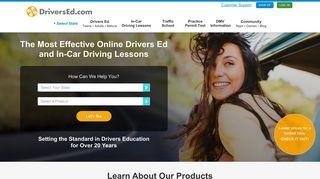This screenshot, taken from the DriversEd.com website, features a central image of a young woman walking with her hair partially covering her face. Despite this, she has turned her head slightly and is smiling. Below the image, there is a rectangular text box prompt asking, "How can we help you?" with several drop-down menus available for selection.

At the top of the screenshot, white text reads, "The most effective online drivers ed and in-car driver lessons." Further down, in black text, the phrase "Learn about our products" is displayed. The top navigation bar includes multiple drop-down menu options, including "Drivers Ed," "In-Car," and "Community," although some options are difficult to read due to the image's low resolution and size.

In the lower right-hand corner, an orange circle contains a message icon, suggesting a chat or help feature. On the left side of the screen, a prominent orange button labeled "Let's Go" invites users to take action. Overall, the screenshot captures the website's user-friendly interface designed to assist visitors in accessing drivers education resources.